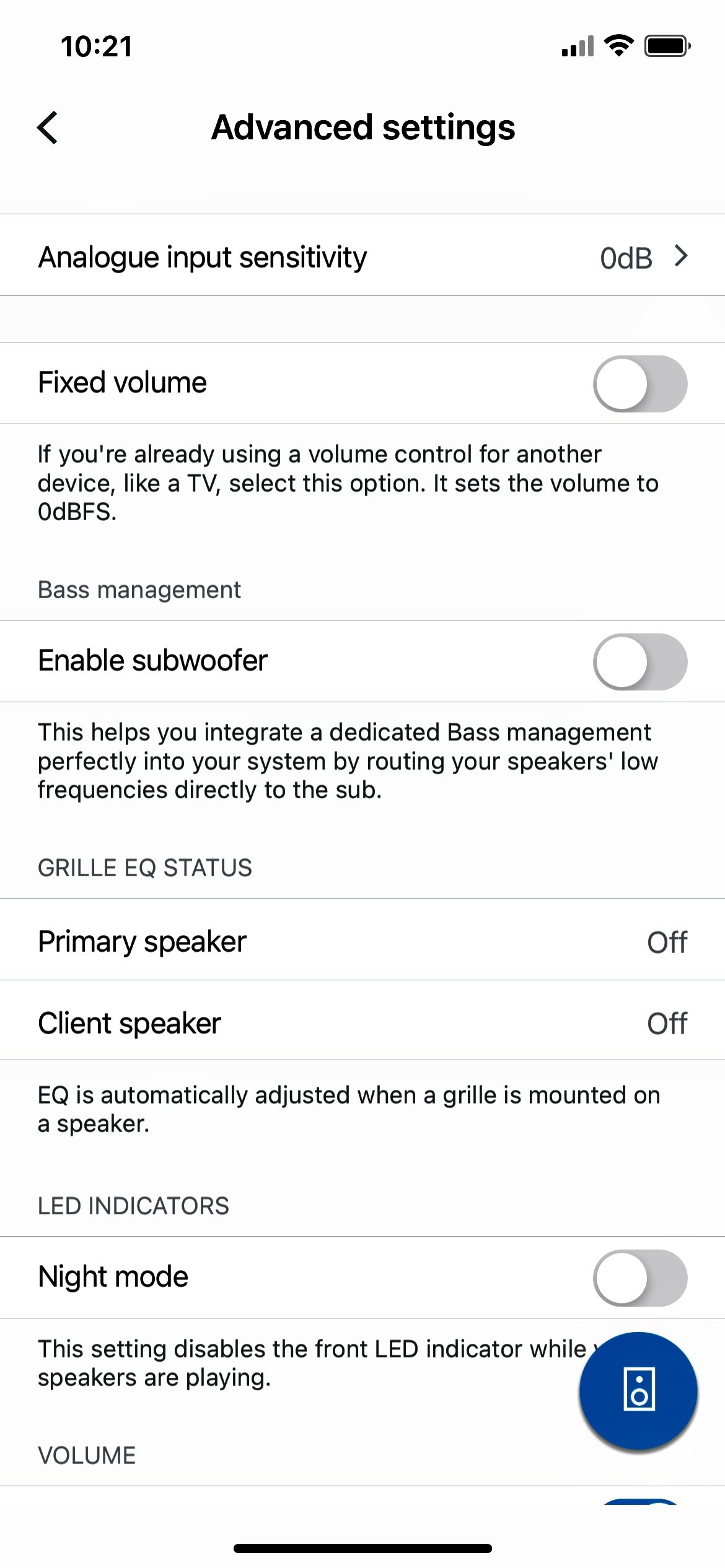In the screenshot, the top right corner displays the battery icon, Wi-Fi signal strength, and phone signal strength, with the phone signal at two out of four bars while the battery and Wi-Fi are fully charged. On the top left, the current time is shown as 10:21. Centered at the top is the "Advanced Settings" label with a leftward arrow. Below this, "Analog Input Sensitivity" is displayed with "0 dB" to its right. 

The next line reads "Fixed Volume," accompanied by an oval-shaped toggle switch that can be set to "On" or "Off." A message underneath recommends selecting this option if another device, like a TV, already utilizes volume control. Further down, "Enable Subwoofer" is indicated with a similar oval toggle switch, explaining that this helps manage bass by directing low frequencies directly to the subwoofer for improved system integration.

In the middle of the image, it mentions "Grill EQ Status." Finally, at the bottom is "LED Indicators," followed by "Night Mode" with an oval toggle. The accompanying note states that enabling this setting will disable the front LED indicator while the speakers are in use.